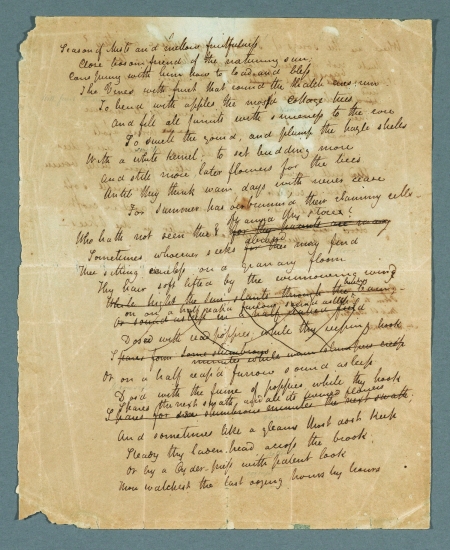The photograph features an aged, handwritten letter on what appears to be leather parchment that has turned a light brown color with time. The text, penned in cursive, is largely illegible due to its small size. The letter is in portrait mode and displayed against a dark gray backdrop, highlighting its cream-colored texture. The letter shows significant signs of wear, with portions torn out from the top left, left edge, bottom left, and top right, where a triangular section appears worn away. The double-sided nature of the letter allows writing from the reverse side to faintly show through. The content is organized into several paragraphs, with some sentences and an entire paragraph crossed out in the center. The opening words seem to say "season of" followed by an unreadable word. The letter has areas with scribbles and X's, indicating changes or redactions made by the original author.